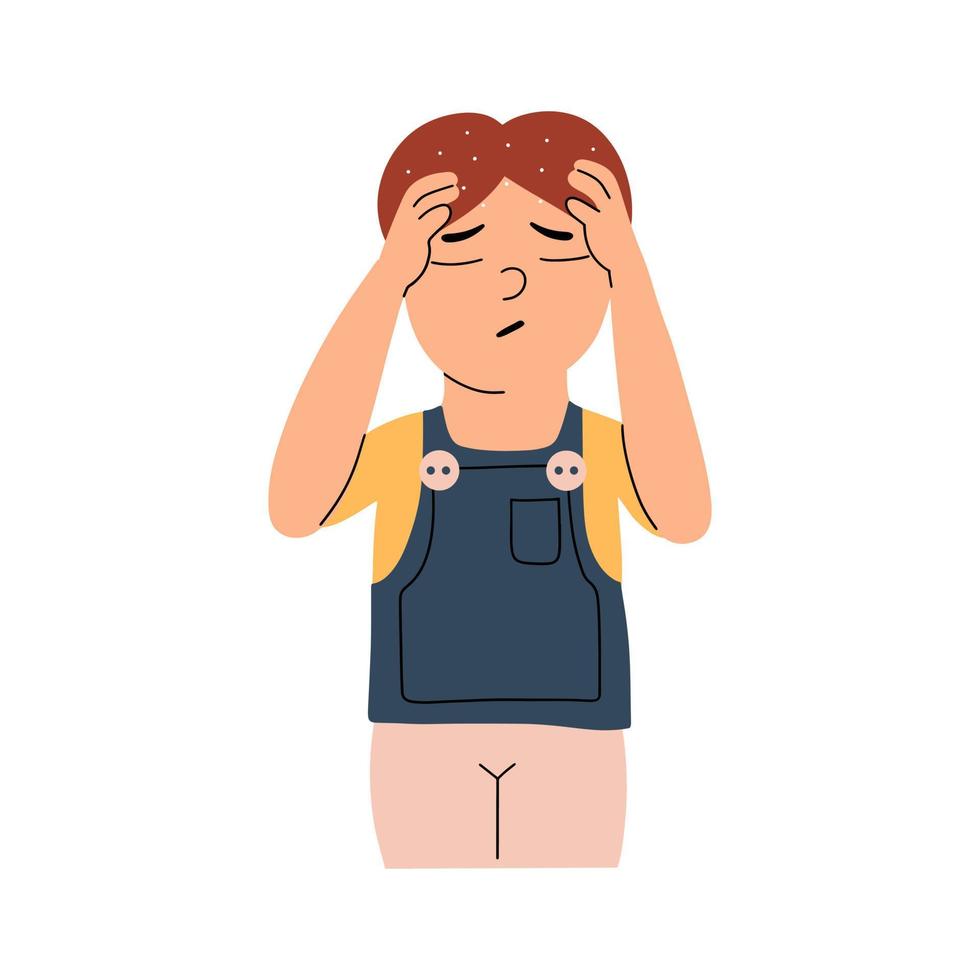This image is a simple, computer-generated cartoon drawing of a young person, possibly a child or a teenager, depicted on a completely white background. The character features short, reddish-brown hair with white specks scattered throughout, suggesting a headache or intense thinking. Their eyes are closed, and they exhibit a pained or stressed expression, with furrowed brows and a small, downward-curved mouth shaped like a diagonal line. 

The character's hands, each showing three fingers, are raised to their temples, emphasizing their discomfort or concentration. They are dressed in a yellow t-shirt and wear blue denim overalls or a smock that covers the top half of their body. The overalls are secured by two white buttons near the neckline and also feature a pocket. The lower half of the character appears either nude or covered in a very light, almost flesh-colored material, with a black, Y-shaped line hinting at the separation of legs.

The overall style of the illustration is minimalistic, focusing on simple lines and basic shapes to convey the scene.